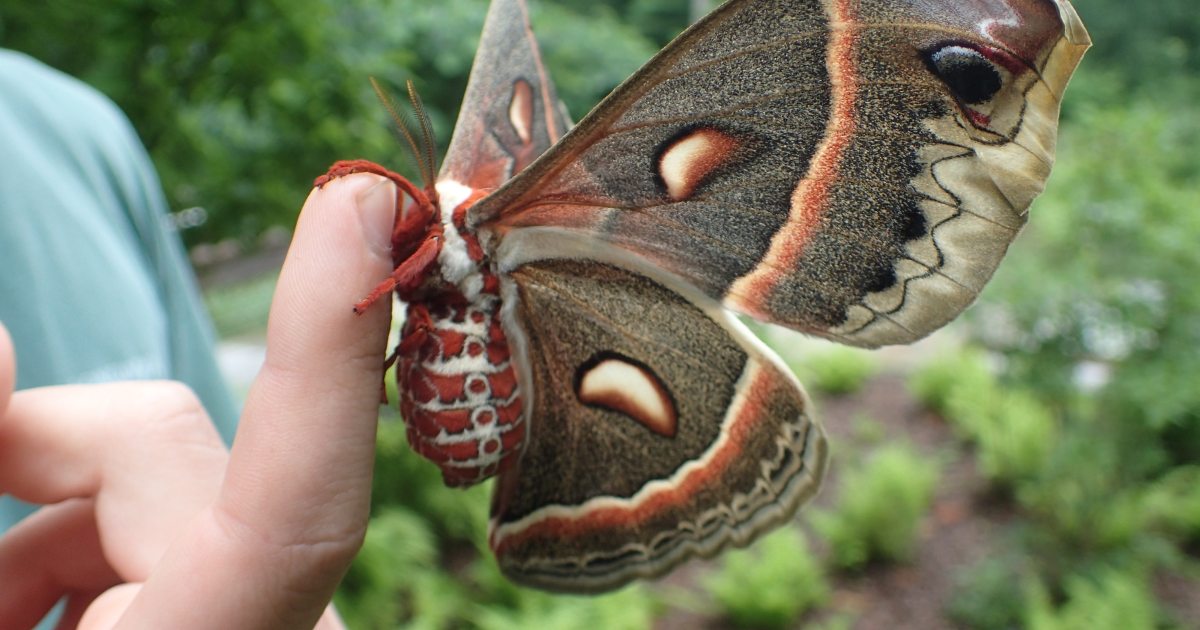This image captures an extremely detailed close-up of a large, fat-bodied moth perched on the raised index finger of a fair-skinned person. The backdrop features an out-of-focus mix of green foliage and a light blue section of the person's shirt on the left side. The person's other fingers are held back, making the moth the focal point. The moth's body is adorned with distinct bands and spots of reddish-brown and white, and it has striking red legs. Its antennae are feathered and appear quite fuzzy. The moth's wings, predominantly visible on the left side, are a blend of brown and gray with a dusty, fuzzy texture, and they feature a light tan edging. There is a prominent rust-colored vertical band and a few false eye spots, including one black and two white ones on each side. The intricate patterns on the wings include a boomerang-like cream-colored shape and are detailed further with rust, cream, and black edging. The moth's vivid coloration and distinctive features are displayed clearly, making it a remarkable and magnified portrait.